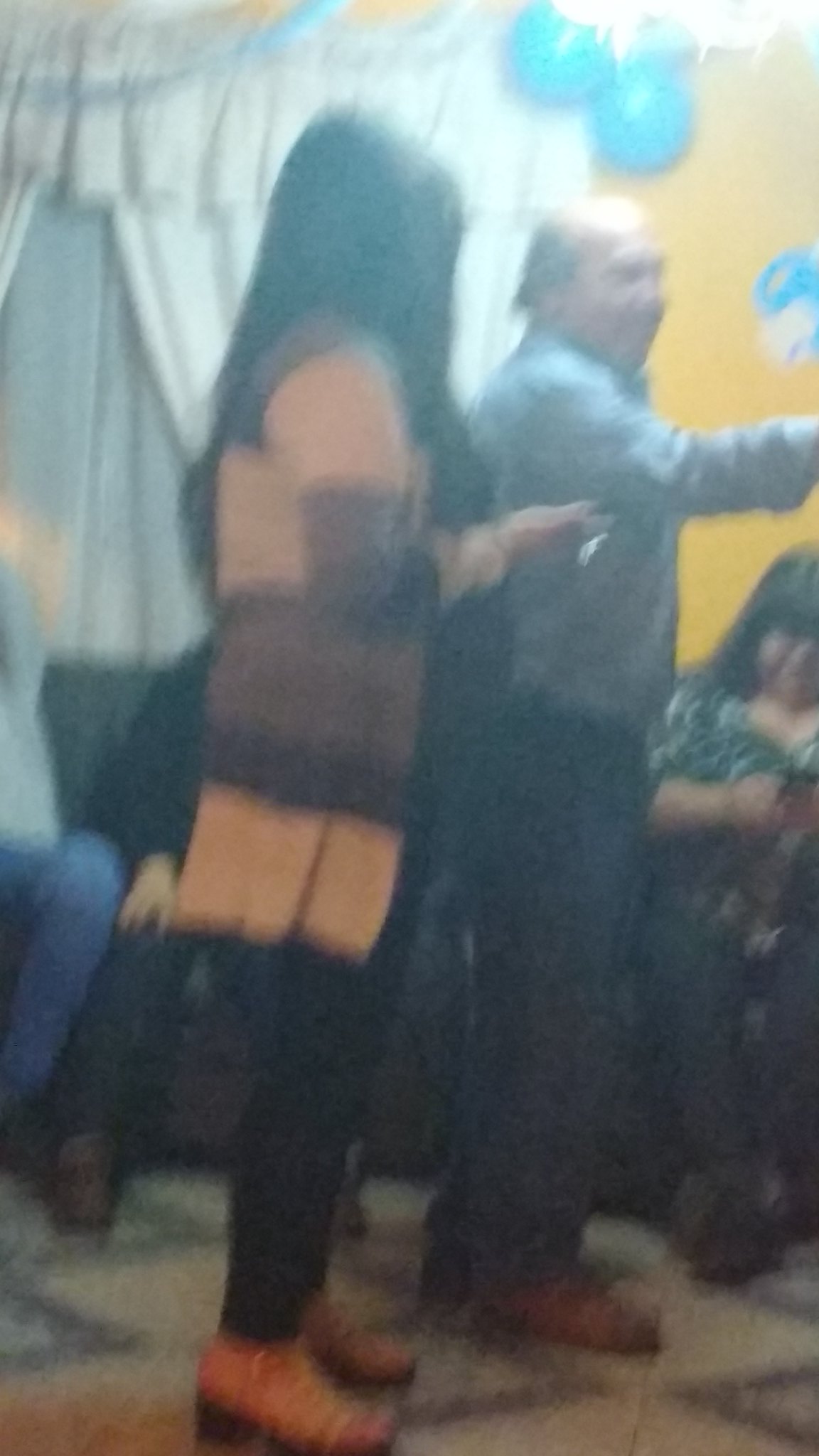This vibrant indoor party scene captures a lively moment amidst cheerful decorations. Set against a yellow wall adorned with blue balloons and white drapes, the photograph reveals a cozy setting with five individuals. A couch is positioned against the curtained backdrop, where two people are partially visible, showing only their legs and one hand. 

To the right side of the couch, a heavy-set woman with brown hair, clad in a green top, is engrossed in her phone. The focus shifts to the forefront where a white male and a female stand facing right. The man, dressed in blue jeans and a blue shirt, is animatedly pointing towards something off-screen. The woman, attired in a tan and brown blouse paired with black pants, gazes attentively at him while holding her own phone. The image captures the essence of social interaction and festive decor, highlighting the warmth and engagement of the party atmosphere.